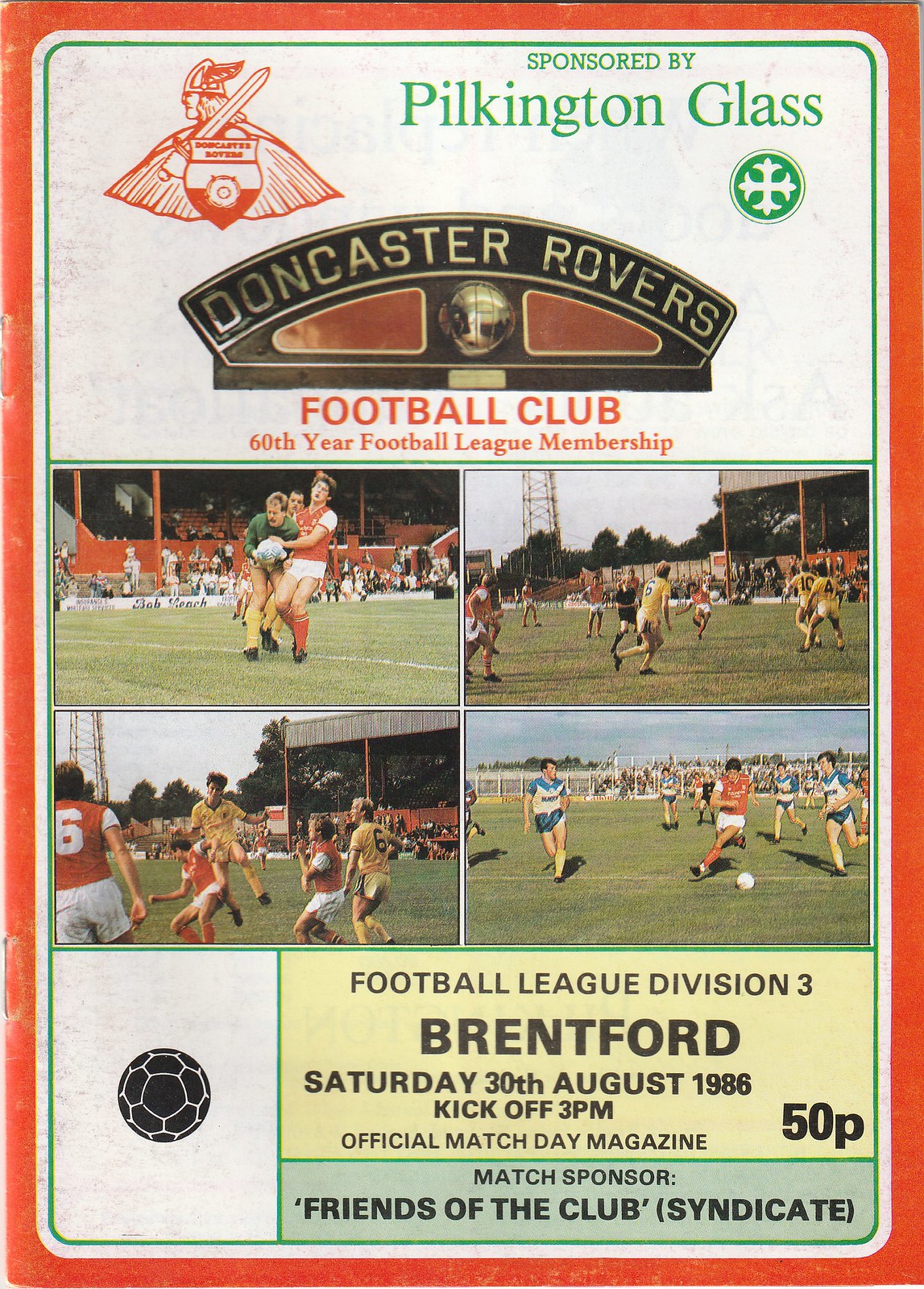This is a detailed photographic-style front page of a soccer program commemorating the Doncaster Rovers Football Club's 60th year of Football League membership. The program is sponsored by Pilkington Glass, whose name is prominently displayed in green text alongside a logo of a Celtic cross. In the top left corner, there is a logo depicting a Viking holding a sword with a shield that reads "Doncaster Division."

The layout features four photos arranged in quadrants: 
- The top left image captures a dynamic moment with a man in an orange and white jersey battling a man in a blue jersey for possession of the ball.
- The top right showcases two full soccer teams on the field, highlighting a player attempting a kick.
- The bottom left image shows an intense action shot with a player leaping into the air amid a crowd.
- The bottom right image features a man in a red jersey and white pants vigorously racing towards the ball, accompanied by blue-and-white-clad opponents.

Below these images, a yellow box provides key match details: "Football League Division III, Brentford, Saturday 30th of August, 1986, kickoff 3pm. Official match day magazine, 50 pence." Beneath this section, a gray or green rectangle states, "Match sponsor, Friends of the Club, Syndicate."

The bottom left corner is adorned with a graphic of a black soccer ball, tying the entire design together.